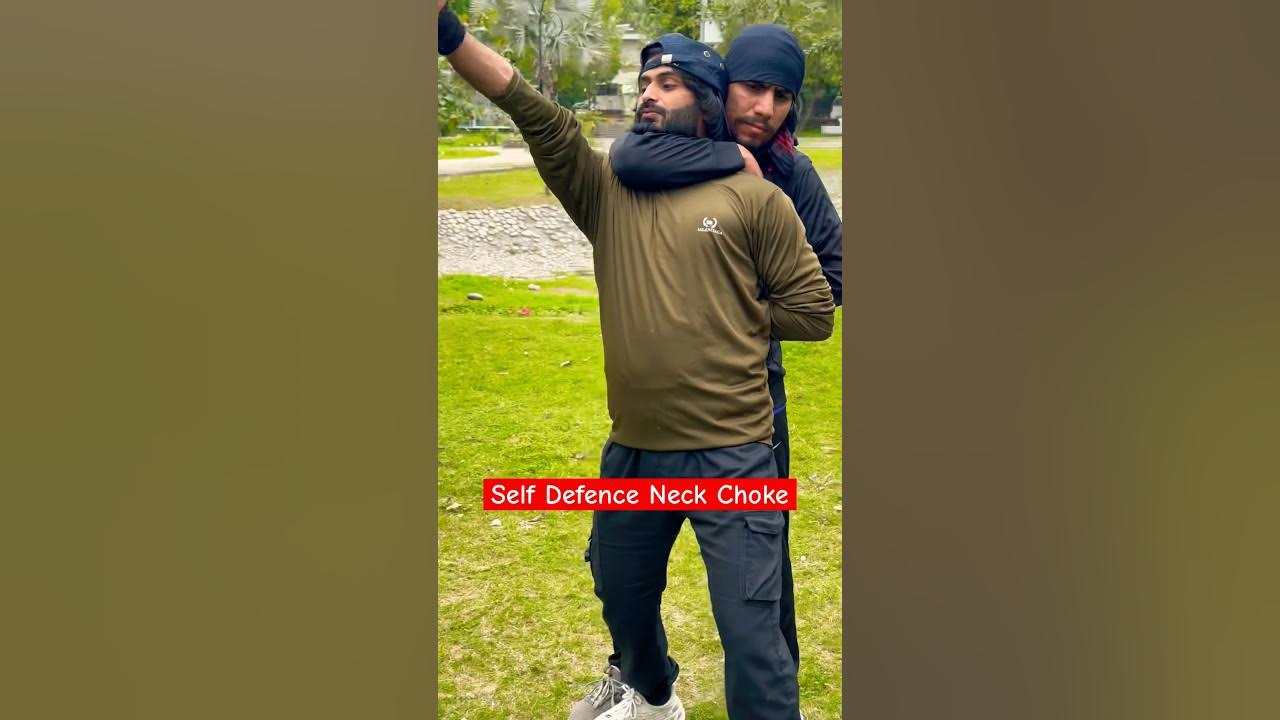In this detailed photograph, two men are demonstrating a self-defense move known as the "self-defense neck choke" in an outdoor grassy field with trees and houses in the background. The man in the back, who has tan brown skin and is dressed in a hoodie, has his arm wrapped around the neck of the man in front. The man in front, characterized by darker skin and a dark brown or black beard, is wearing a backwards baseball cap and an olive long-sleeve shirt. He also has his left arm held behind his back by the man applying the choke, leaving his right arm extended in front of him. Both men are wearing blue jeans and the man in front has white sneakers. Notably, the scene is set against a dark olive green background in a portrait orientation, captured in a representational realism style. At the bottom third of the image, a red rectangular banner with white text prominently displays the words "self-defense neck choke."